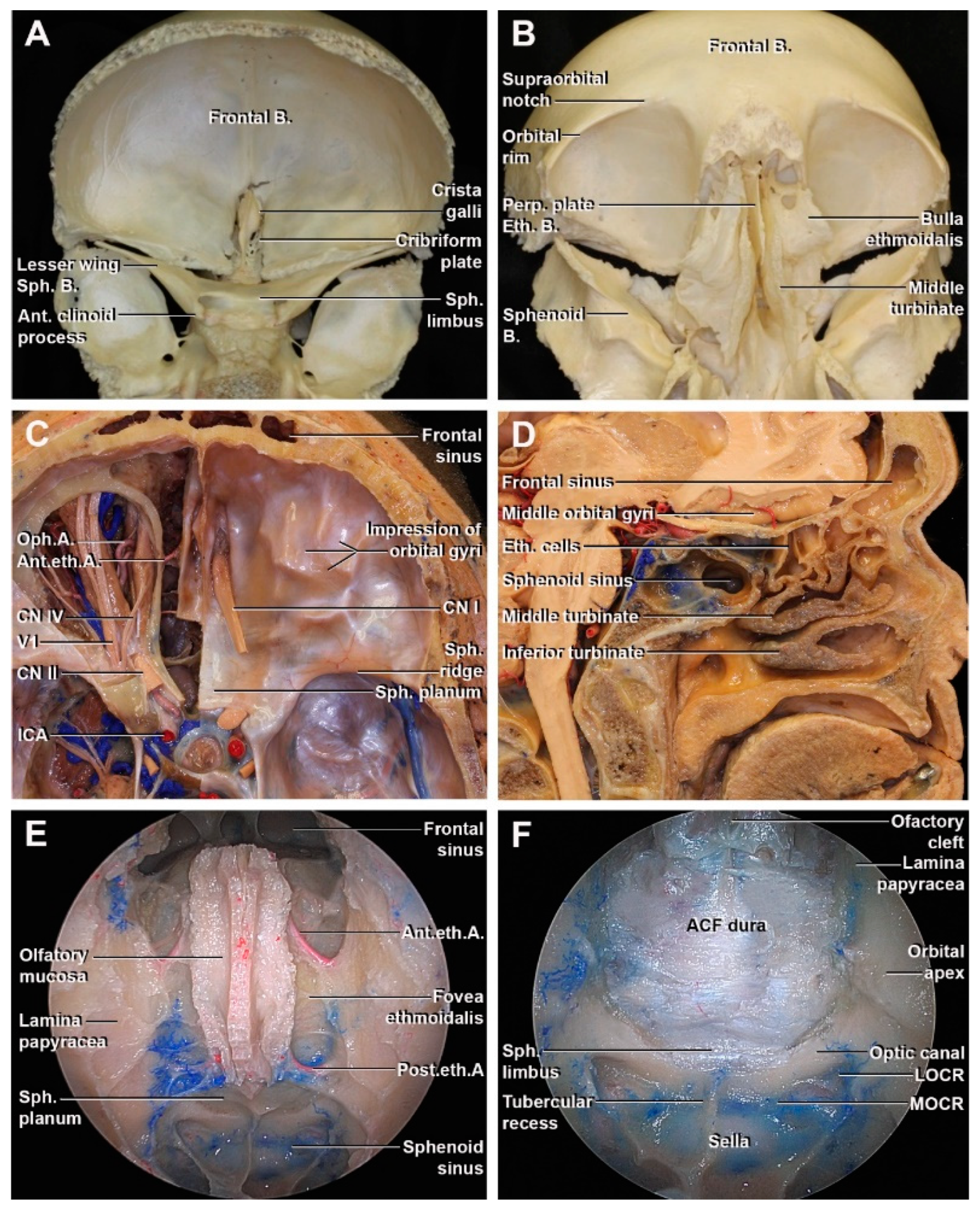This detailed medical poster features a grid of six images labeled A through F, each depicting various anatomical sections and structures of the skull. Image A shows a frontal view of the skull, highlighting the frontal bone and associated structures labeled as "frontal B." Image B also presents a frontal view, adding detailed labels such as the orbital rim, orbital notch, and sphenoid. Image C offers an intricate interior cross-section, revealing the frontal sinus, orbital impression, and essential vessels and tendons. Image D provides a deeper cross-sectional view of the sinus area, while Image E presents an angle view emphasizing the olfactory mucosa and the associated anatomical features. Finally, Image F focuses on the dura mater within the anterior cranial fossa, labeled with specifics like "ACF dura." Overall, this poster meticulously illustrates the frontal and internal aspects of the skull, including sinuses, eye sockets, and vital anatomical landmarks.